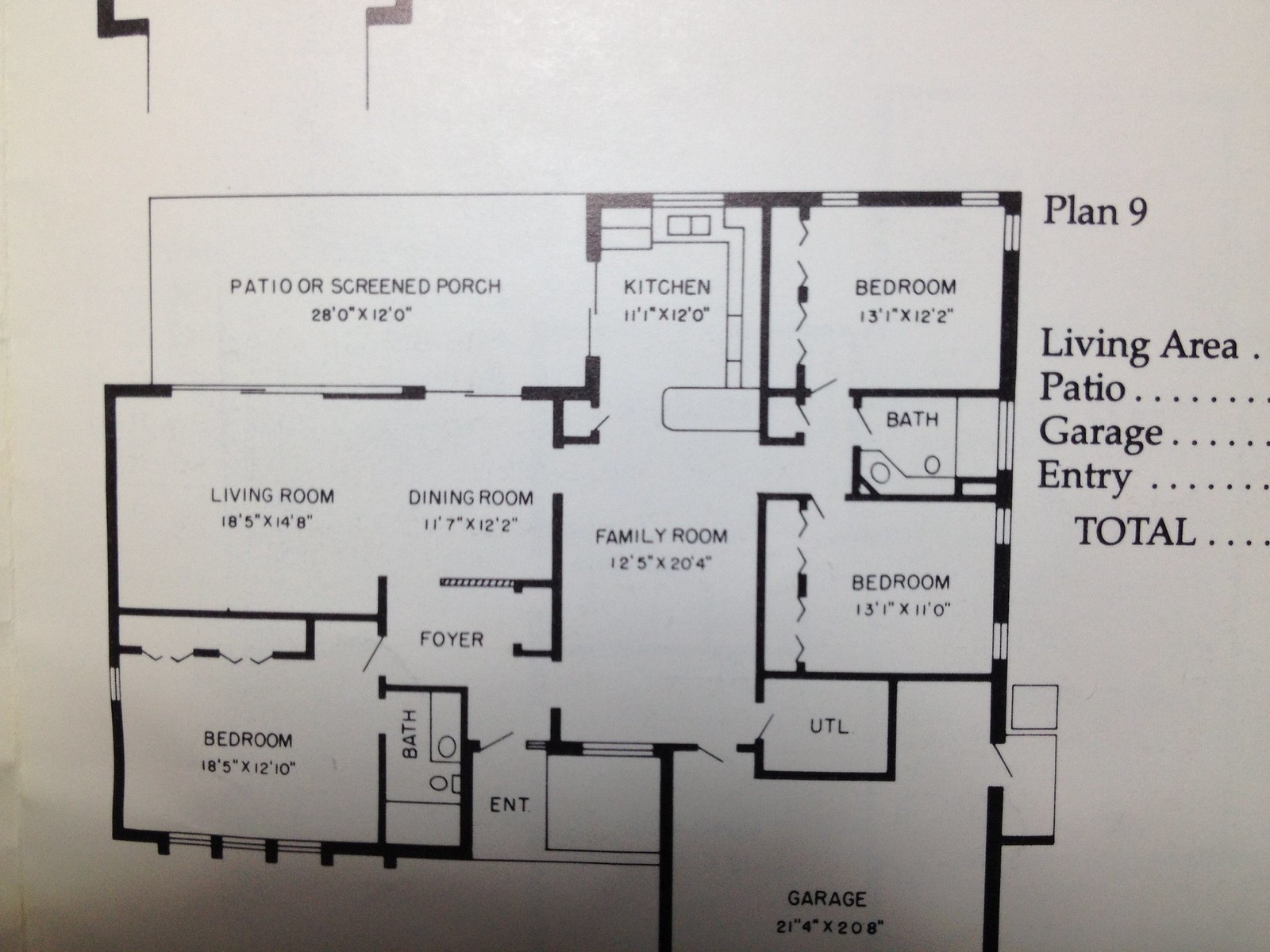A detailed black-and-white floor plan of a spacious house, depicting the essential layout of various living quarters. The blueprint includes labeled rooms such as bedrooms, dining rooms, bathrooms, and a kitchen, each with their dimensions specified in feet and inches. It features symbols indicating doors, closets, windows, and entryways such as the main entrance and foyer. While the bathroom details like the bathtub, toilet, and sink are illustrated in a simplified manner, there's no indication of where most of the furniture is placed in the other rooms. Despite the apparent size of the house, the total square footage or area is not provided.